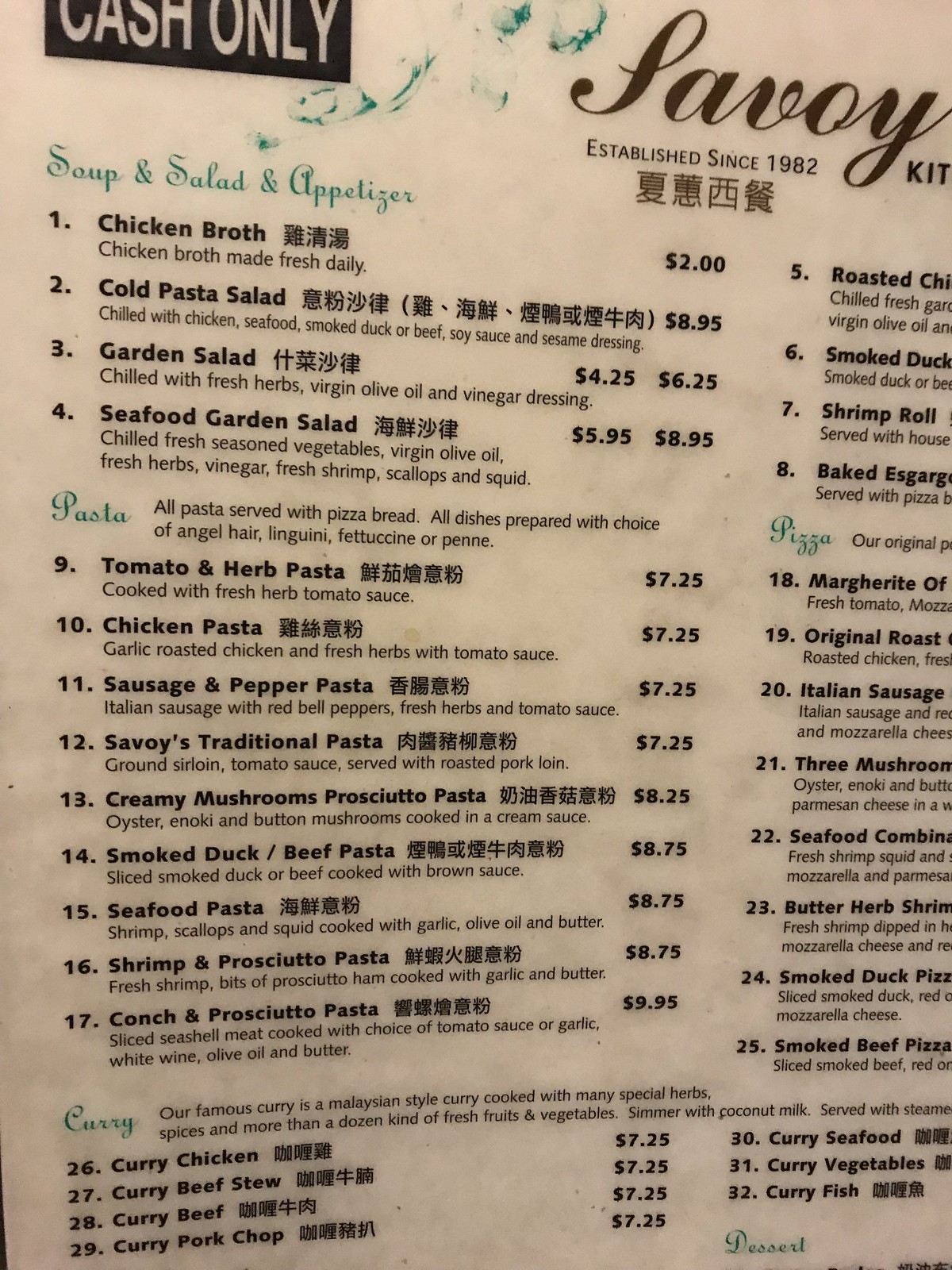This vertical close-up image showcases a detailed view of the Savoy restaurant's menu against a tan background. In the upper left corner, a black rectangle with transparent areas highlights the "Cash Only" policy of the establishment. The menu, established in 1982, displays an elegant layout with black text in varying font sizes to distinguish different sections and items.

At the top of the menu, the Soup and Salad section lists various options with prices ranging from $2 to $8.95. Below that, the Appetizers section teases the diverse selection available to diners. The next prominent section focuses on Pasta, featuring eight to nine choices such as Tomato and Herb Pasta, Seafood Pasta, and Conch and Progetti Pasta, demonstrating the restaurant's versatile culinary expertise. Following these, a list of curry dishes is presented, each priced at $7.25.

This detailed close-up image captures the essence of the Savoy kitchen's menu, emphasizing its long-standing tradition and diverse offering.